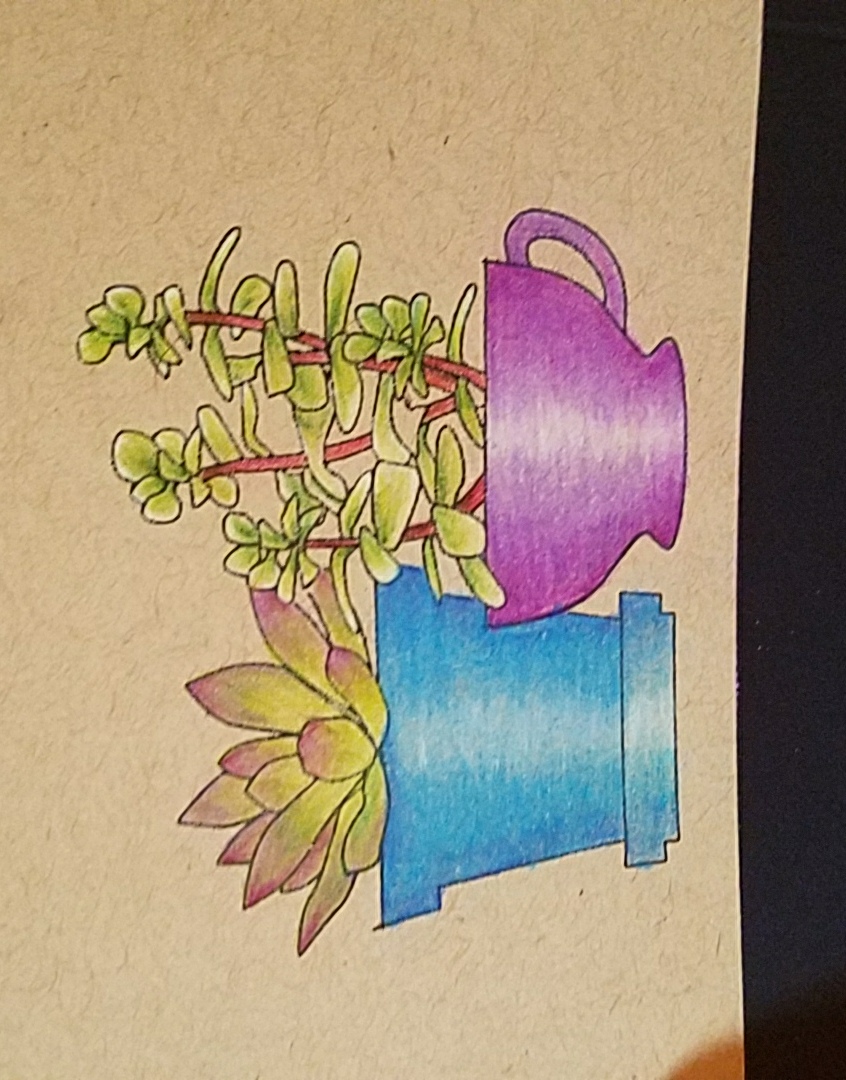This image is a color photograph of a pen and ink drawing on a textured watercolor or thick art paper, which gives the artwork a tactile, almost fibrous appearance with tiny lines resembling fine hairs woven into the surface. The drawing features a low-set coffee cup shaded in hues of purple, positioned on the right side of a square-shaped flower pot. Emerging from this pot is a cactus or succulent plant characterized by soft, squishy leaves. The plant lacks distinct stems and is shaded with a rich palette of purple, blue, light green, pinkish-purple, and light brownish-pink hues. The overall composition blends intricate line work with subtle, harmonious color shading to create a visually striking and detailed botanical illustration.